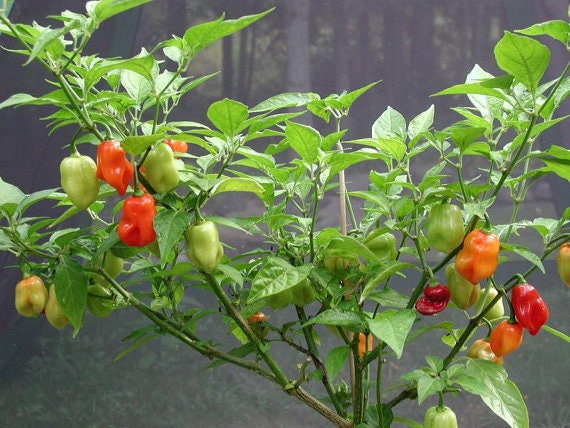A close-up photograph captures a vibrant pepper plant with thin, bright green stems branching out in multiple directions. The plant is adorned with lush green leaves and a variety of small, oblong-shaped peppers resembling habaneros. The peppers exhibit a range of colors, from light green to orange, yellowish-orange, red, and dark red, creating a vivid and colorful display. The background is blurry and muted, possibly due to fog or mist, giving hints of a forest with trees, green bushes, and what appears to be a gray cement slab at the bottom. The natural, serene background contrasts with the sharp focus and vivid colors of the pepper plant in the foreground.